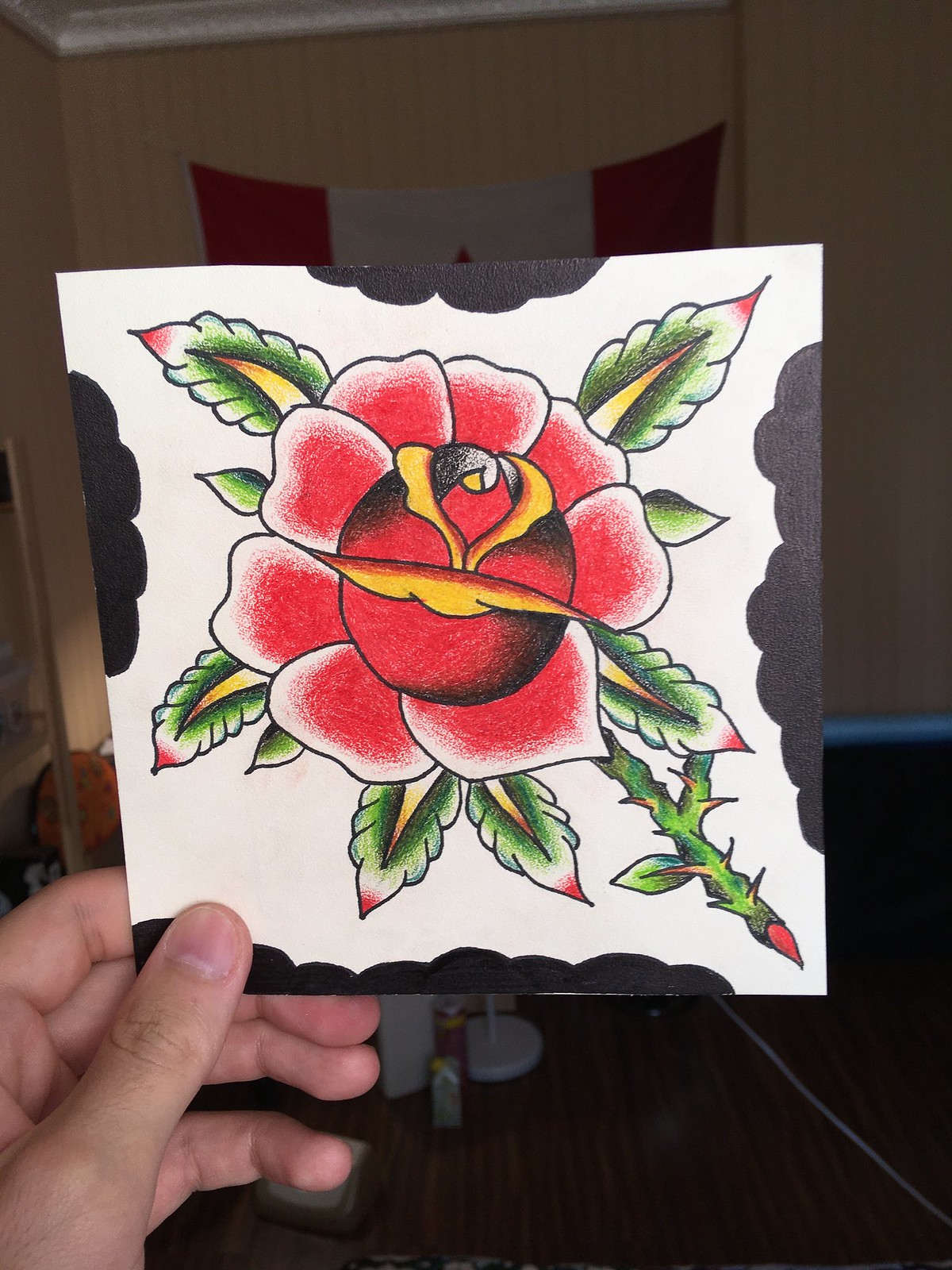A detailed piece of art is held in the left hand of an anonymous person. The hand, visible with a thumb and fingers, firmly grips the bottom left corner of the square, white paper. The edges of this paper are adorned with four distinctive cloud-like borders, each sketched in black. Dominating the center of the artwork is a vibrant drawing of a rose, its petals an alluring mix of pink and red hues. The rose's green stem extends diagonally towards the bottom right, accentuated by menacing thorns. The accompanying leaves, also green, bear a spiky texture with reddish-pink thorns further emphasizing their form. Expertly applied shadows, in black and white, add depth and contrast to the overall composition.